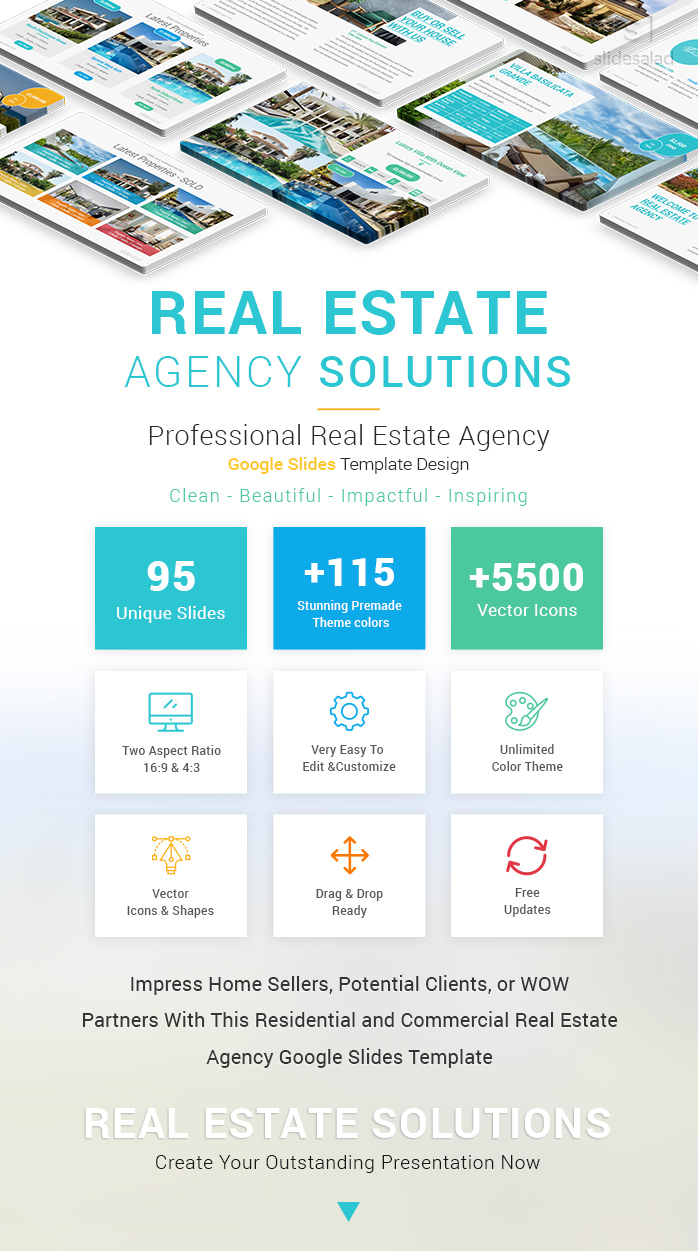The image displays a screenshot or screen capture featuring a promotional material for a Google Slides template named "Real Estate Agency Solutions." The top section has a grayish background with various texts in distinct colors, including "Real Estate Agency Solutions" in aqua blue, "Professional Real Estate Agency" in black, "Google Slides" in gold, "Template Design" in black, and "Clean and Beautiful, Impactful and Inspiring" in teal.

Above these texts, there is a banner showcasing several images that appear to be real estate listings with various amenities. Below the banner, there are several colorful square boxes. The first box is teal with white text that reads "95 Unique Slides." The second box is blue with white text that likely says "115 Theme Colors," though the exact phrase is difficult to discern. The third box is green with white text that says "5500 Vector Icons."

Further down, there is a row of six white boxes, each featuring black text and colored icons. The first box states "Two Aspect Ratio" with a teal computer icon. The second box, with a blue cogwheel, mentions something related to configuration or settings, potentially "Color Themes." The third box highlights "Vector Icons and Shapes" with an orange icon. The fourth box, containing text about easy customization and possibly stating "Drag and Drop Ready," has orange arrows. The fifth box mentions "Free Upgrades" coupled with magenta arrows. The sixth box may contain a promotional statement targeting home sellers, potential clients, or partners, emphasizing that this Google Slides template is perfect for making impressive presentations.

The bottom section reiterates the template's name "Real Estate Agency Solutions" in white text on a more visually appealing background, ending with "Create Your Outstanding Presentation Now" in black text combined with a teal arrow pointing forward.